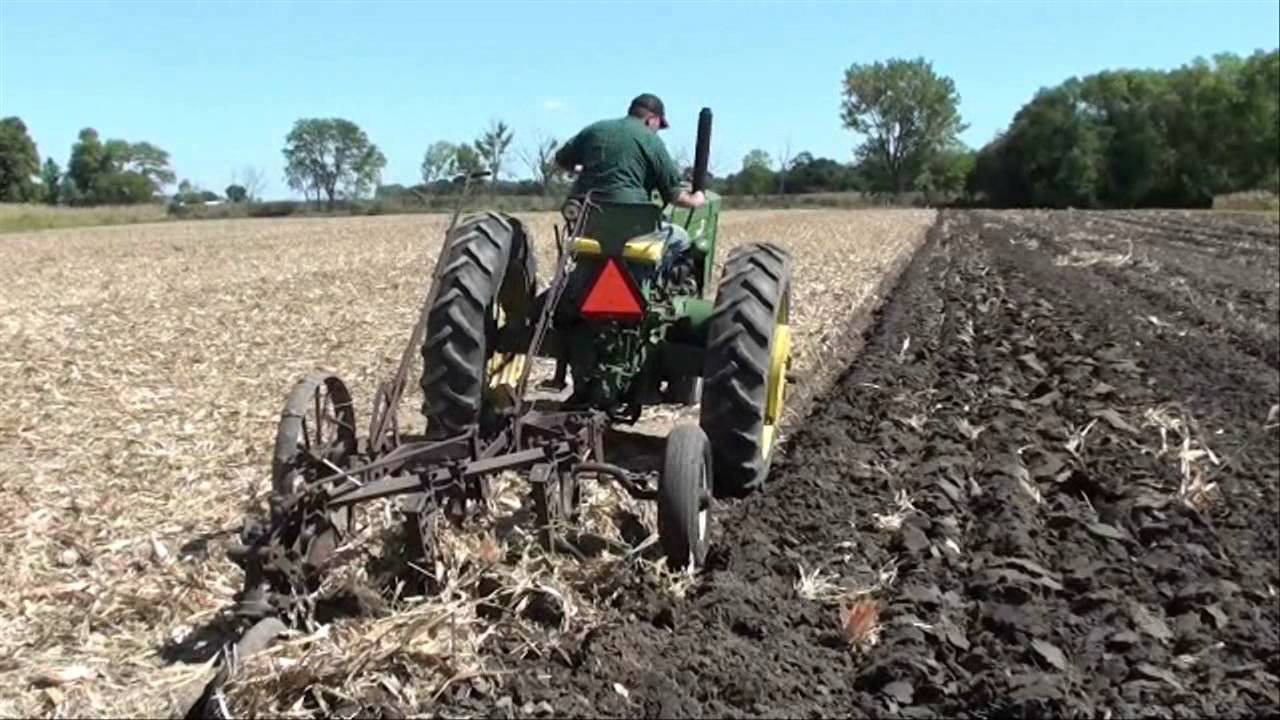In this detailed outdoor photograph, a farmer is captured mid-task as he tills his field with a John Deere tractor. The scene is set under a clear blue sky with just one visible cloud, framed by trees with sparse leaves, indicating a late spring day, possibly around May or early June. The farmer, dressed in a green long-sleeve shirt and a black baseball cap, is driving away from the camera, emphasizing the back view of both him and the tractor.

The tractor, characteristic with its iconic green color and large rear wheels with yellow rims, is fitted with a tiller attachment at the back, suggested by the orange triangular slow-moving vehicle emblem. As the farmer maneuvers through the field, the left side remains unplowed, visibly marked by dry, yellowish dirt and old corn stalks. In contrast, the right side of the field showcases the freshly tilled soil, dark and ready for planting. This picturesque, action-filled shot vividly encapsulates a day in the life of a dedicated farmer preparing his land for the next planting season.